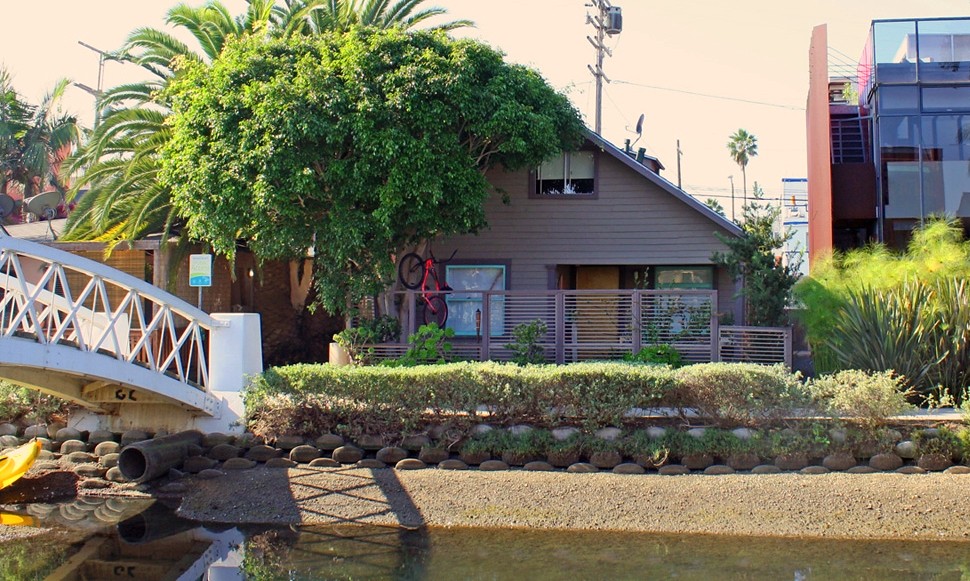This is a color photograph that captures a richly detailed scene of a neighborhood featuring a two-story light brown house with a gray roof. The house, prominently positioned in the center, has brown window frames and a front doorway. On the roof, a satellite dish is pointed leftward. Adjacent to the house, on the left side, stands a very large green tree with a palm tree just behind it. 

The front of the house features a small walkway lined with rocks on a lower sloped area, leading to what appears to be either a drainage ditch or a small river running from right to left at the bottom of the photograph. This waterway is brown in color, flanked by an embankment of sand or gravel.

Behind the light brown house is a slotted fence, offering a glimpse of a red bicycle hanging from a tree in the backyard. To the left side of the image, partially visible, is a white footbridge. Adjacent to this, there is another house—constructed from stone or brick—with a gray roof. To the right of the central house is an office building with glass windows.

The background features a gray sky dotted with telephone poles and another palm tree, encapsulating the tranquil and varied elements of this residential scene.